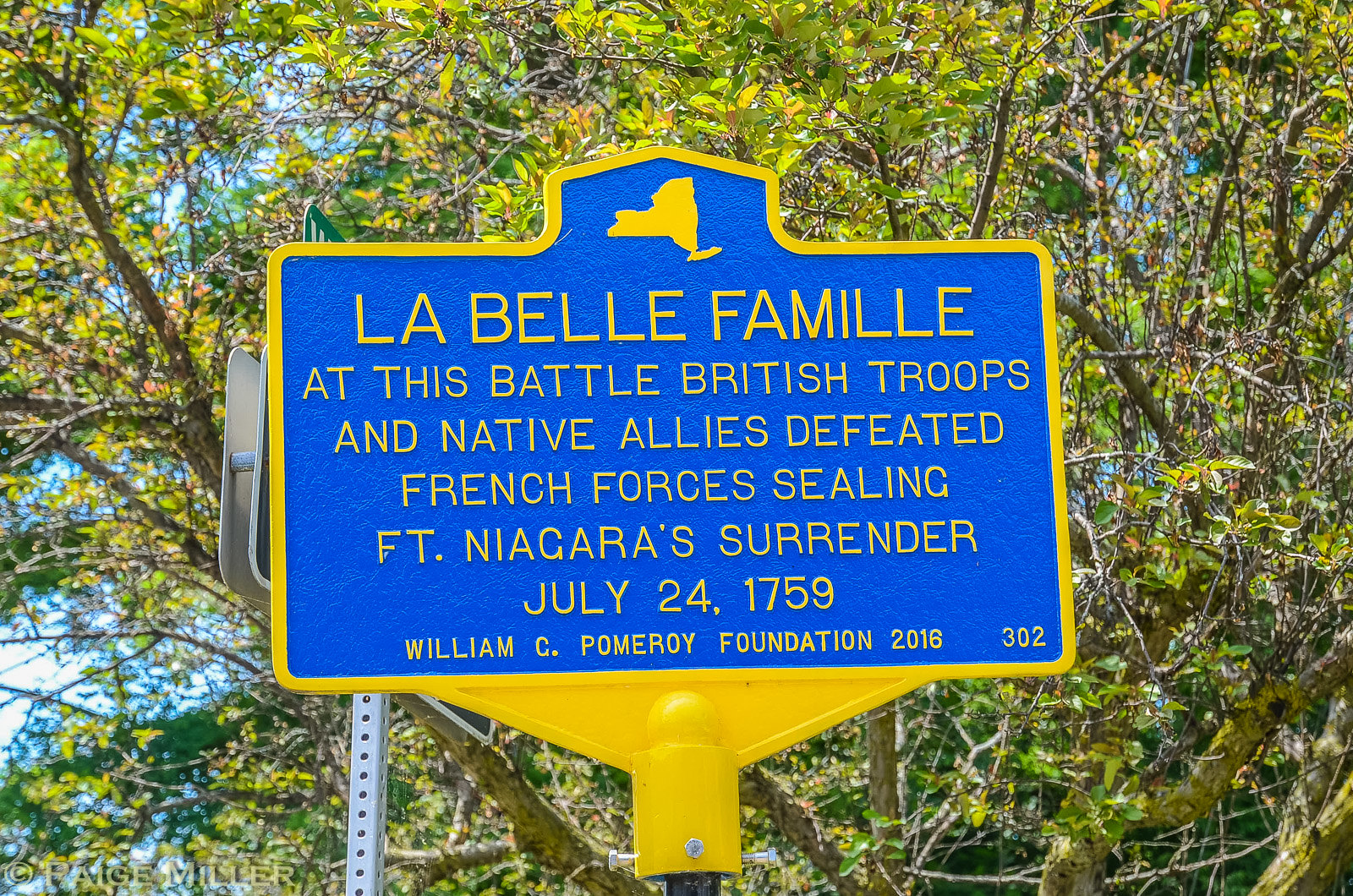The photo, taken in the daytime, depicts a prominently featured historical sign positioned outdoors. The sign, mounted on a perforated silver pole, is bordered in a vivid yellow with a dark blue background, making it stand out against the surrounding greenery of trees and glimpses of the blue sky. The sign, crowned by a pointed top that bears a yellow logo resembling a map, contains yellow, all-caps text that reads: "La Belle Famille, at this battle British troops and native allies defeated French forces sealing Fort Niagara's surrender, July 24th, 1759. William C. Pomeroy Foundation, 2016." At the bottom right, the number "302" is also inscribed in yellow. The overall composition includes branches with green leaves further framing the sign, and partially obscured in the background is another post or pole. The bright sunlight enhances the clarity and color contrasts in the image.